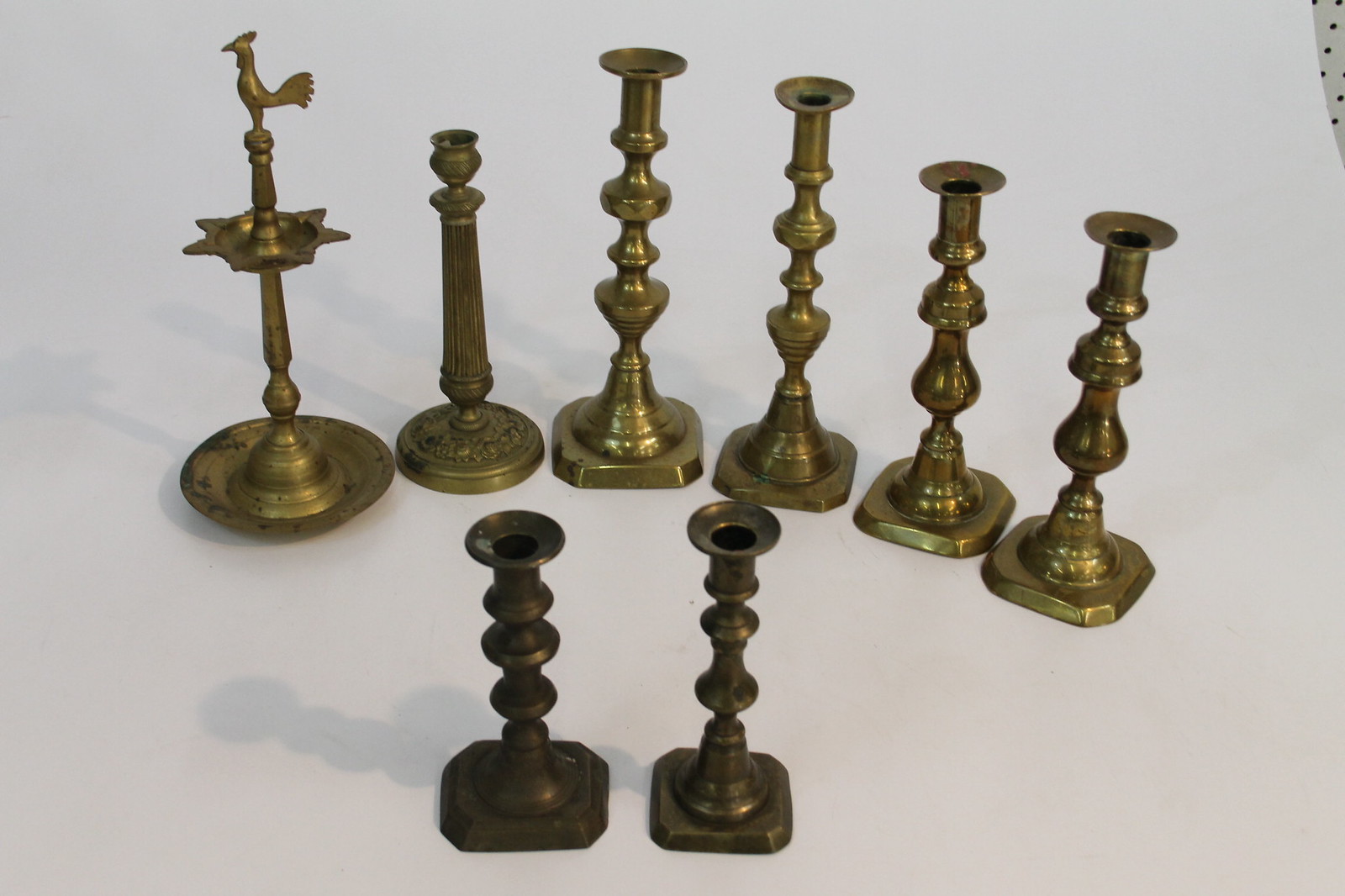The photograph captures a collection of eight distinctive candle holders arranged on a light orchid cloth that covers a table, with a glimpse of black and white polka dot material in the top right corner. The base of the setup appears to be a white backdrop that extends from the floor to the wall, providing a clean, neutral background. 

In the foreground, there are two shorter, tarnished brass candle holders with a spiral design, exhibiting a blackish patina while still retaining some shine. These two stand apart from the six larger ones in the back, which are arranged in an arch from left to right. 

On the far left is a unique candle holder with a large circular base and an intricate design featuring a rooster perched on top, facing left. This candle holder is copper-colored with a star-like pattern midway up the stem. Next to it is another slender candle holder with a ribbed, column-shaped structure and a simple, cylindrical form.

The four candle holders to the right of these two are similar in style, each positioned on a flat, square base with rounded edges. They are characterized by a series of narrow and bulging sections, creating a visually interesting, bubbled effect. Two of these are slightly shorter, while the other two are taller. Their surfaces exhibit less tarnish and more of a yellowish brass hue compared to the darker, smaller holders in the front.

Overall, the collection showcases a variety of heights and detailed designs, with the taller ones forming a backdrop to the shorter, more worn pieces in the front. The overall effect is enhanced by the thoughtfully arranged placement and contrasting finishes, creating a visually cohesive and interesting display.